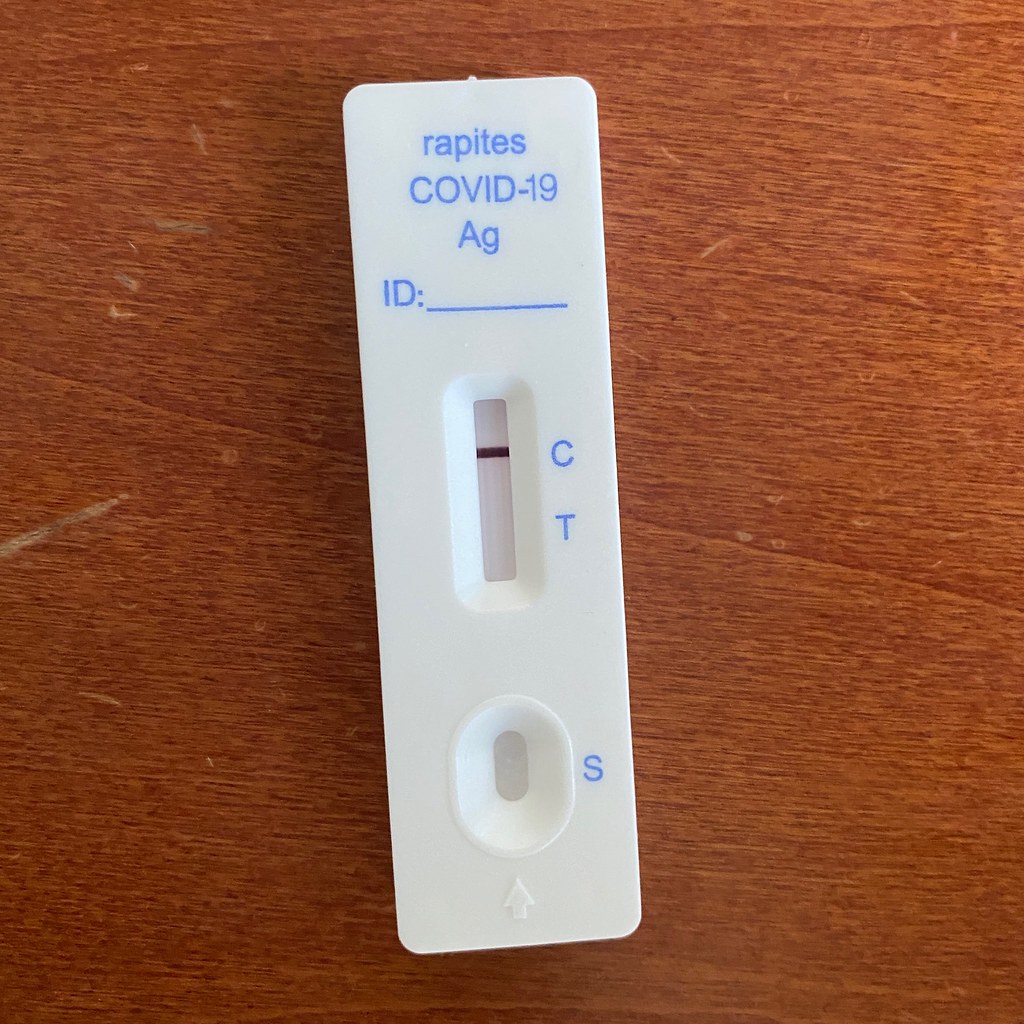The image features a small, white plastic COVID-19 test kit labeled "Repetiz COVID-19 AG." The label includes a large 'A' followed by a small 'G'. An 'ID:' field with a blank line is provided, presumably for inscribing a name or other identifier. The test kit has markings for 'C' (control), 'T' (test), and a small slot labeled 'S', with an arrow embossed on it, indicating where the test sample should be placed. A dark line appears next to the 'C', which likely signifies a control marker. The inscriptions on the test kit are in blue letters, while the line near the 'C' is black. The kit is placed on a wooden table with a golden brown, slightly scuffed surface, adding a rustic backdrop to the image.